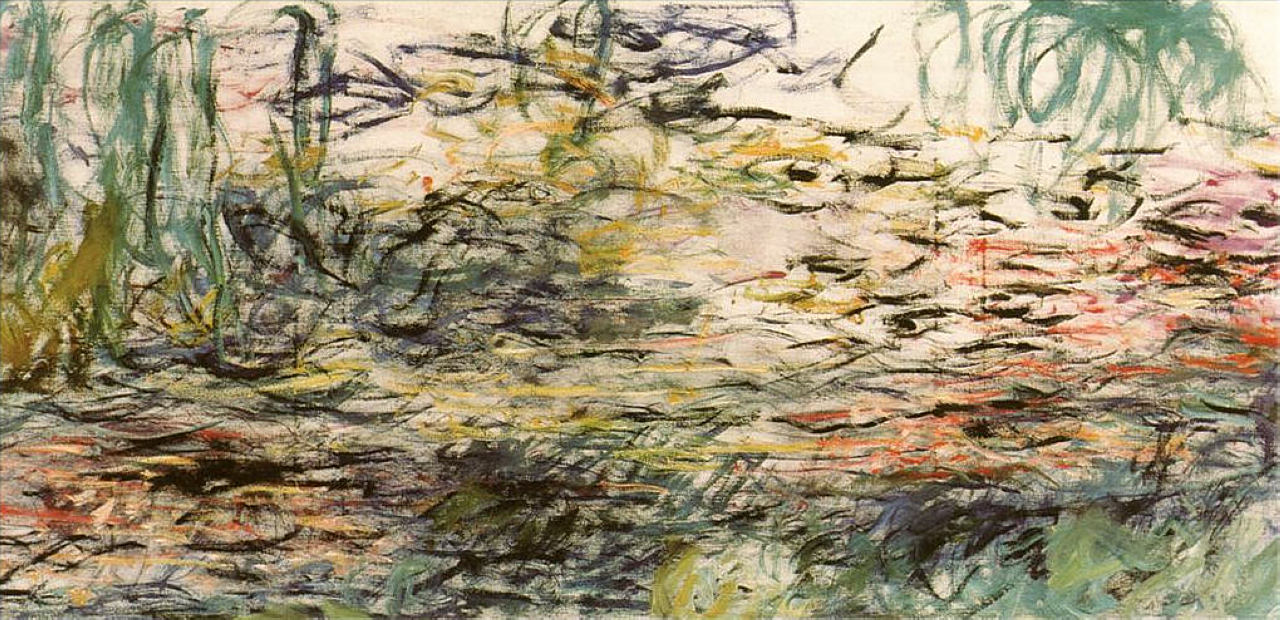This horizontal rectangular image is a modern abstract painting that can be interpreted in various ways. Dominated by shades of green—including light green, dark green, and teal—the image possibly depicts a swampy area or a river scene filled with plant life and hints of water. The bottom portion of the painting features what appears to be grasses, water, or muddy terrains with a mix of tans, browns, and touches of orange. The upper right side showcases lighter shades, which might suggest the presence of tree branches and the sky, while the upper left side contains wisps of green, likely representing plants growing upwards and some brown marks that resemble driftwood or fallen logs. The foreground is denser with prominent black lines and dark-green streaks that evoke the image of weeds protruding from the water. This thick, intricate layer of colors—ranging from yellow and red to black—creates a textured, almost murky water scene filled with indistinct objects like fish or eyes lurking within. The background is predominantly white with streaks of tan, suggesting clearer water as the scene recedes. This captivating and intricate painting draws viewers in with its complex interplay of colors and floating forms, offering multiple interpretations and an immersive visual experience.